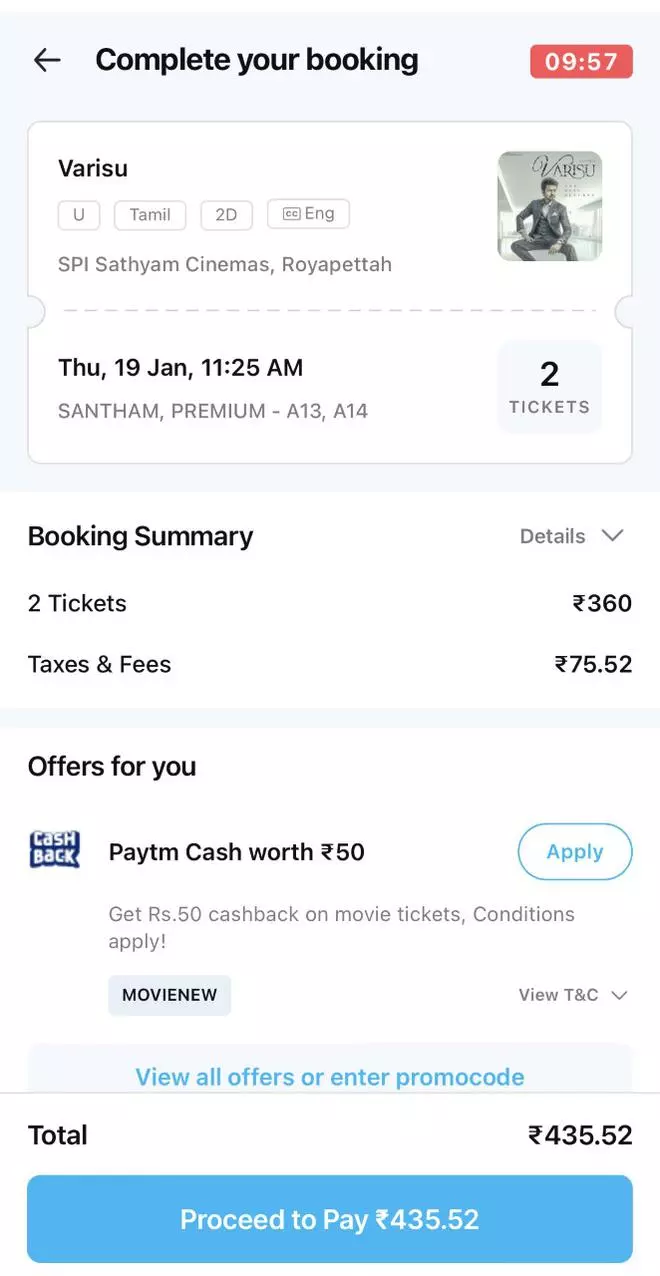The image showcases a mobile phone screen displaying a movie ticket booking interface, presumably from India, as indicated by the use of rupee currency. The top section of the screen is predominantly gray, featuring bold black text that reads "Complete your booking" accompanied by a black arrow pointing to the left. Adjacent to this is a countdown timer set at 9 minutes and 57 seconds, suggesting a 10-minute window to finalize the booking.

Within this gray box lies an image of a movie ticket, along with details such as "Varasu U Tamil 2D CC," which signifies the movie "Varasu" in Tamil with closed captioning in English. The cinema is identified as "SPI Santham Cinemas Royapetha" and includes a picture of a man in a suit, presumably a character from the movie "Varasu." Below these details is a dotted line separating the information fields. The bottom section specifies the showtime: "Thursday, January 19th, 11:25 a.m.," with seats numbered "Santham Premium - A13, A14" and indicates "Two tickets" in black ink.

Moving down into a white area, the title "Booking Summary" appears in bold text, with a corresponding details dropdown menu on the right side. This section lists the cost for "Two tickets at 360 rupees" and "Tax and fees at 75.52 rupees." A light gray bar below these details introduces an offers section with the text "Cashback" next to a blue and white icon. It highlights a specific offer: "PayTM cash worth 50 rupees - Get 50 rupees cashback on movie tickets, conditions apply," alongside an oval "Apply" button. 

Following this is a "Movie New" section in a gray box with a dropdown for viewing terms and conditions labeled "View T&C." Another gray box below this offers further options to "View all offers and enter promo code," displayed in aqua text. The total amount for the booking sums to "435.52 rupees," with an aqua button reading "Proceed to pay 435.52" in white text.